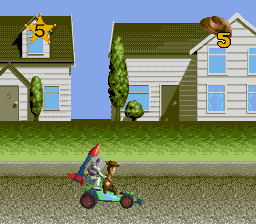This is a screenshot from a Toy Story-themed video game. The image captures a small, vibrant scene where iconic characters Woody and Buzz Lightyear are riding on a toy car, zooming down a street adjacent to the curb. In the background, there’s a gentle grassy hill followed by two suburban houses, adding depth and context to the setting. The upper-left corner of the screen displays a star icon marked with the number five, likely indicating a score or level. Similarly, the upper-right corner features an icon of Woody's hat, also accompanied by the number five, suggesting a counter or status indicator relevant to Woody's character. The whimsical scene is bursting with the nostalgic charm of the beloved Toy Story franchise, encapsulated within the dynamic world of the video game.